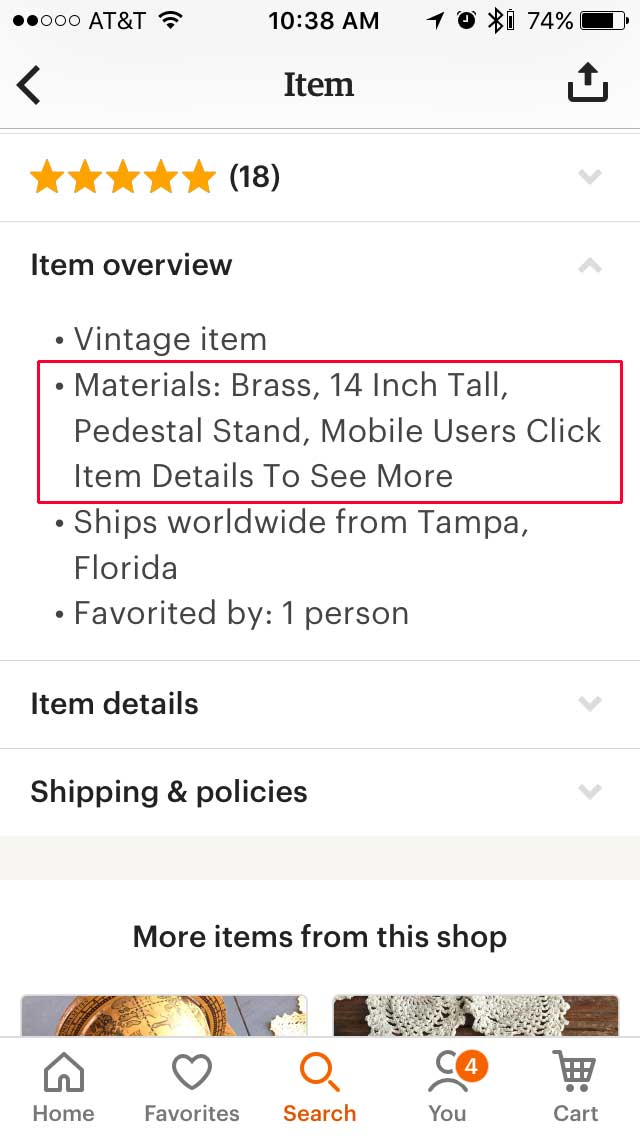The image depicts a digital product listing page on a white background. At the top, there is a blue status bar indicating the network carrier as AT&T, the time as 10:38 AM, and a battery level at 74%. Below this, a navigation bar features a left arrow and the word "Item," followed by an icon of an open box with an upward arrow.

The listing shows a 5-star rating with the number 18 beside it. An expandable section titled "Item Overview" indicates the product is a vintage item. Below this, a red box displays specific details: "Materials: Brass," "14-inch tall pedestal stand," and a note for mobile users to click for more details. Shipping information includes "Ships worldwide from Tampa, Florida," with a note that the item is "Favorited by one person."

Further down, there are sections labeled "Item Details" and "Shipping and Policies," each with a down arrow indicating expandable content. A segment titled "More Items from This Shop" shows partially visible images of two additional products.

At the bottom of the page, a navigation bar includes icons labeled "Home," "Favorite," "Search," "You" (featuring a red dot with the number 4), and "Cart."